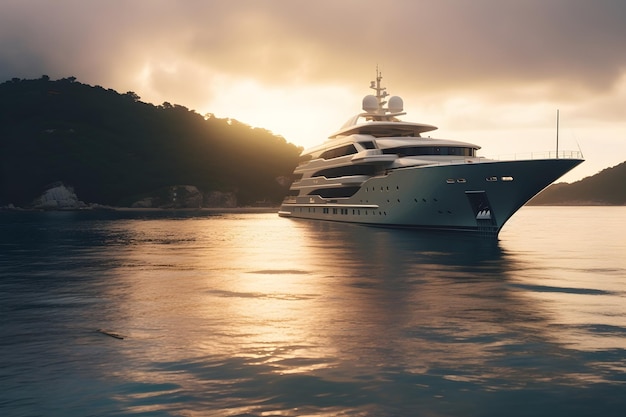The image features a large, four-level yacht prominently positioned near the center, slightly angled so the front extends to the far right. The yacht appears to be sailing in calm, reflective waters that occupy the lower half of the scene, creating gentle light ripples. Behind the yacht, a shoreline is visible, framed by a tree-lined forest that extends from the middle left to the far right, providing a lush backdrop. Above this, a sky filled with numerous clouds dominates the top third of the image, with the sun partially breaking through, casting a grayish-bluish hue across the scene. The overall color palette includes bright white from the yacht, light yellow from the sun, and varying shades of blue, gray, and hints of black. Notably, the scene lacks any text or human presence, focusing purely on the serene outdoor setting of the yacht close to the shore.